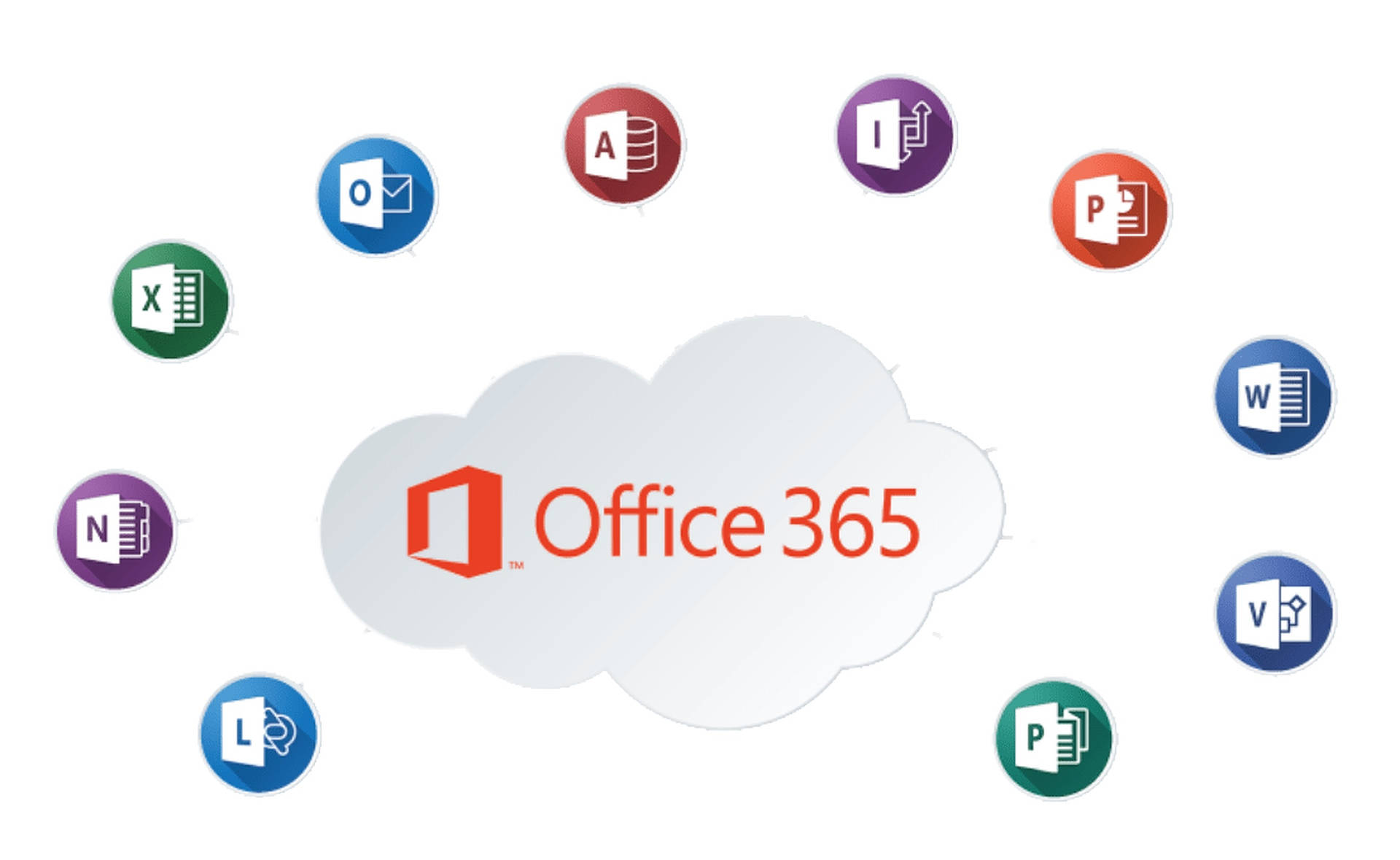**Advertisement for Microsoft Office 365: A Modern Productivity Suite**

The advertisement centers around a prominent cloud graphic emblazoned with "Office 365" in a striking orange-red hue. Encircling this central cloud are various familiar application icons from the Office 365 suite, including:
- **L**: Likely representing Outlook
- **N**: OneNote
- **X**: Excel
- **O**: Outlook for email
- **A**: Access
- **I**: InfoPath
- **P**: Project
- **W**: Word
- **V**: Visio
- A second **P**: Publisher

Each icon represents a key component of the Office 365 offering, though their precise identities may not be immediately clear to all viewers. The layout suggests a comprehensive, integrated suite of tools essential for modern productivity.

This image contrasts the all-in-one simplicity of past versions of Microsoft Office, such as those available in Windows XP, with the subscription-based, segmented approach of Office 365. This transition encapsulates the shift towards cloud-based services and subscription models in contemporary software distribution.